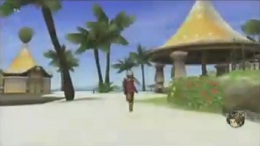A tiny, somewhat blurry image depicts a person in a brown outfit and helmet walking toward the camera on a broad sandy path. In the background, a round gazebo with stone pillars and a pointed roof stands prominently. Surrounding the scene are numerous palm trees, adding a tropical vibe to the setting. Further in the distance, the vast blue ocean can be seen under a bright blue sky. To the left of the wide path, there's a rectangular building, possibly a residence, crowned with a cone-shaped dome.